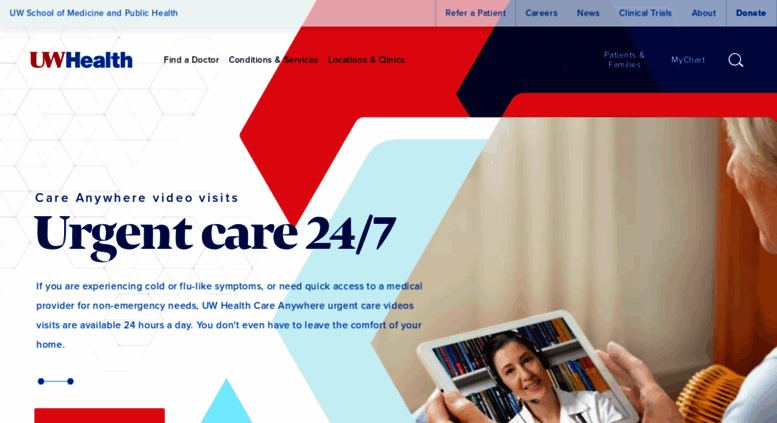**Website Homepage of UW School of Medicine and Public Health**

In the top left corner, the website proudly displays the name "UW School of Medicine and Public Health" in a prominent manner. Below that, in a striking combination of red and blue, it reads "UW Health." Spanning from left to right, the navigation bar includes the options "Find a Doctor," "Conditions and Services," and "Locations and Clinics." These options likely feature drop-down menus to facilitate site navigation and provide a user-friendly experience.

The right side of the page exhibits the same red and blue theme and displays a picture of a hospital at the bottom. On the left side of the image, an arrow points upward, drawing attention to the text "Drive-Thru Convenience." Below this, in smaller font, it states "John Wall Drive-Thru Clinic," followed by a few descriptive sentences.

A light blue arrow and a small circle in the top right section of the page indicate additional clickable options that run across the page, including "Refer a Patient," "Careers," "News," "Clinical Trials," "About," and "Donate." Beneath these options lies a search bar with the "My Chart" feature below it.

In the lower left corner, the webpage features a frontal view of a hospital-like building. The structure, made of concrete with several windows, has a tree in front of it, and the interior lighting is visible, lending a welcoming ambiance to the facility.